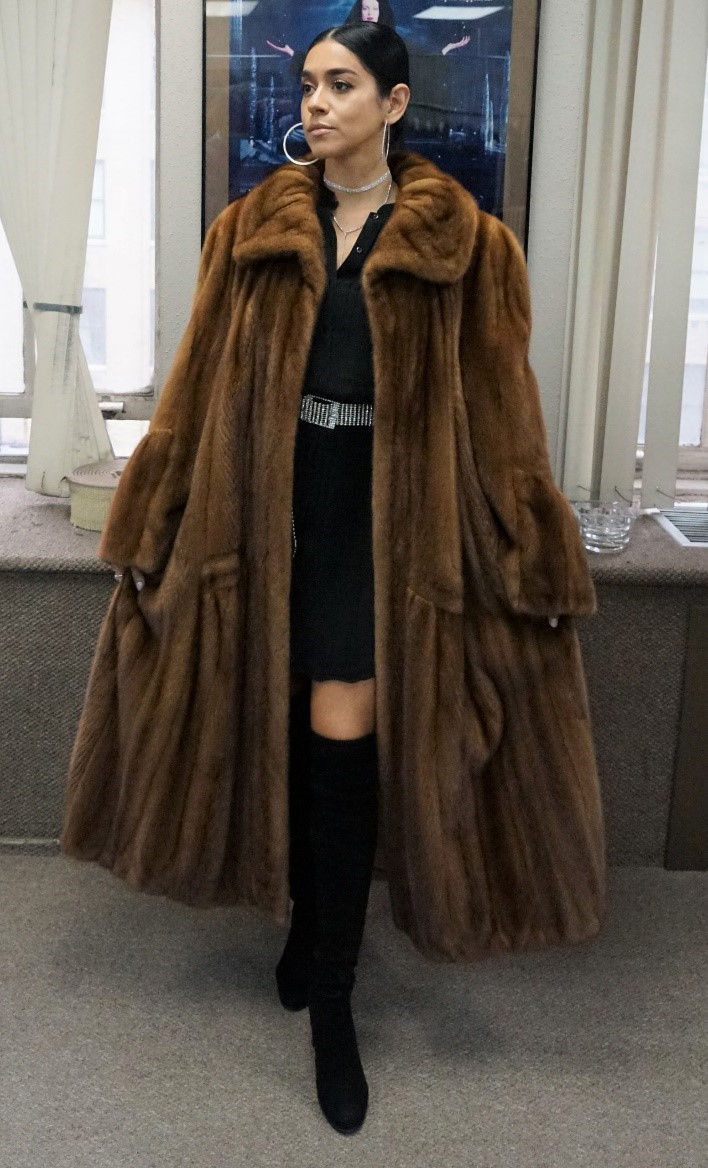The image features a woman standing confidently in the center of a room adorned with brown carpeting and framed by a gray bench and white-curtained windows on either side. She is enveloped in an opulent, dark brown fur coat that extends halfway to her ankles, revealing a black dress underneath, cinched at the waist with a silver belt. The dress stops just above her knee, complementing her knee-high black boots. Her attire is accentuated by large silver hoop earrings and a silver choker necklace, along with another necklace adding a touch of elegance. Her glossy black hair is styled back, either in a low ponytail or bun. The woman strikes a poised pose with her arms slightly outstretched, pulling the coat open, while she gazes off to one side with a serious expression. Behind her, the muted tones of the room are punctuated by a dark, glossy photograph, capturing just the top of a woman's face and her outstretched arms, which reflect some of the room's ambiance. Overall, the scene is defined by a palette of browns, blacks, tans, and whites, suggesting a sophisticated and stylish setting.